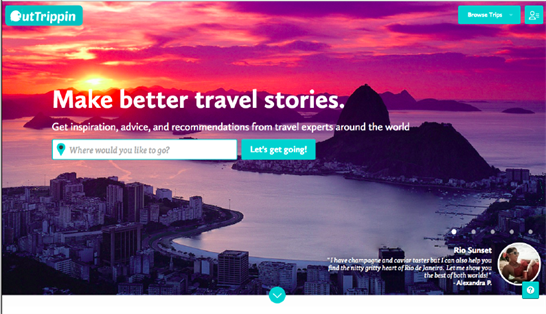The image features a diverse and vibrant travel-themed collage. In the top left corner, a green section labeled "Browse Trips" showcases an extraterrestrial figure, reminiscent of E.T., experiencing a surreal, trippy moment. In the background, a character adorned in shades of red, purple, white, and yellow stands out, exhibiting striking purple claws. 

Dominating the backdrop is a majestic sunset scene with hues of purple and blue reflected in the water, creating a picturesque setting. A prominent sign invites viewers to "Make Better Travel Stories," encouraging them to seek inspiration, advice, and travel insights from around the globe, with the prompt, "Where would you like to go? Let's get going."

A section titled "Rio Sunset" features luxurious elements like champagne and caviar, enhancing the allure of Rio de Janeiro. It promises to reveal both the glamorous and the authentic heart of the city, guided by Alexander Peay. Peay is depicted relaxing in a tree, dangling over the beach, embodying a blend of adventure and leisure.

Towards the bottom, a green square and a central green circle highlight key choices or destinations. The scene transitions to an urban landscape with a densely packed harbor and tall buildings, illustrating the bustling and vibrant urban sprawl.